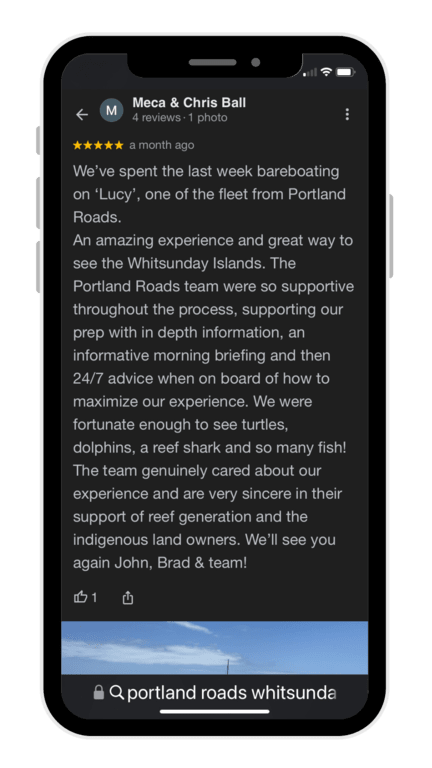The image displays a smartphone screen featuring a review post against a very dark gray background. At the top, the text is in white, while the majority of the post's text is in light gray. The post is authored by "Mecca and Chris Ball," indicated next to a circular grayish-blue icon on the left, which features a white uppercase "M" at its center. An arrow pointing to the left, likely a back button, is also part of this icon. Below their name, there are five bright gold stars indicating a five-star rating, and the review was posted a month ago. The review itself is detailed, praising an amazing experience and the enjoyment of exploring the islands. At the bottom of the screen, there is a partially visible photograph accompanying the review, showing a blue sky with white, fluffy clouds. Additionally, the bottom section contains a search icon, next to which the text "Portland Roads" and "Whitsunda" (spelled "W-H-I-T-S-U-N-D-A") is visible.